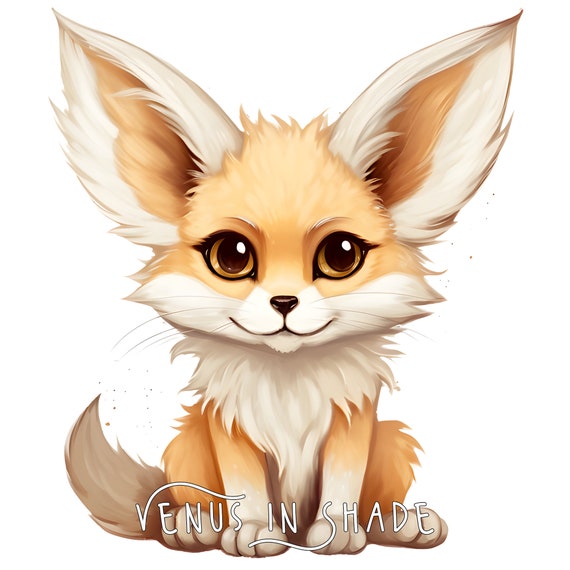This digital drawing features an adorable, small fox with a light tan and white color scheme. The fox is characterized by its large, upright ears, which are tan with white outlines, and a pair of dark brown eyes that shine with a light brown outline. It has a fluffy, brown tail that points to the left, and its fur appears extremely smooth and soft, giving it a lifelike yet cartoonish quality. Its lower face and belly are highlighted with white fur, and it sports a cute, button-like nose. The fox is sitting on a white background, emphasizing its presence. Beneath the illustration, there's white lettering that reads "Venus in Shade," with the letters "V" and "S" artistically designed with long curves, potentially indicating the author or artist's signature. This simple yet detailed drawing, possibly AI-generated or digitally illustrated, belongs to someone skilled in digital art, and it might be a character from a comic book or video game.